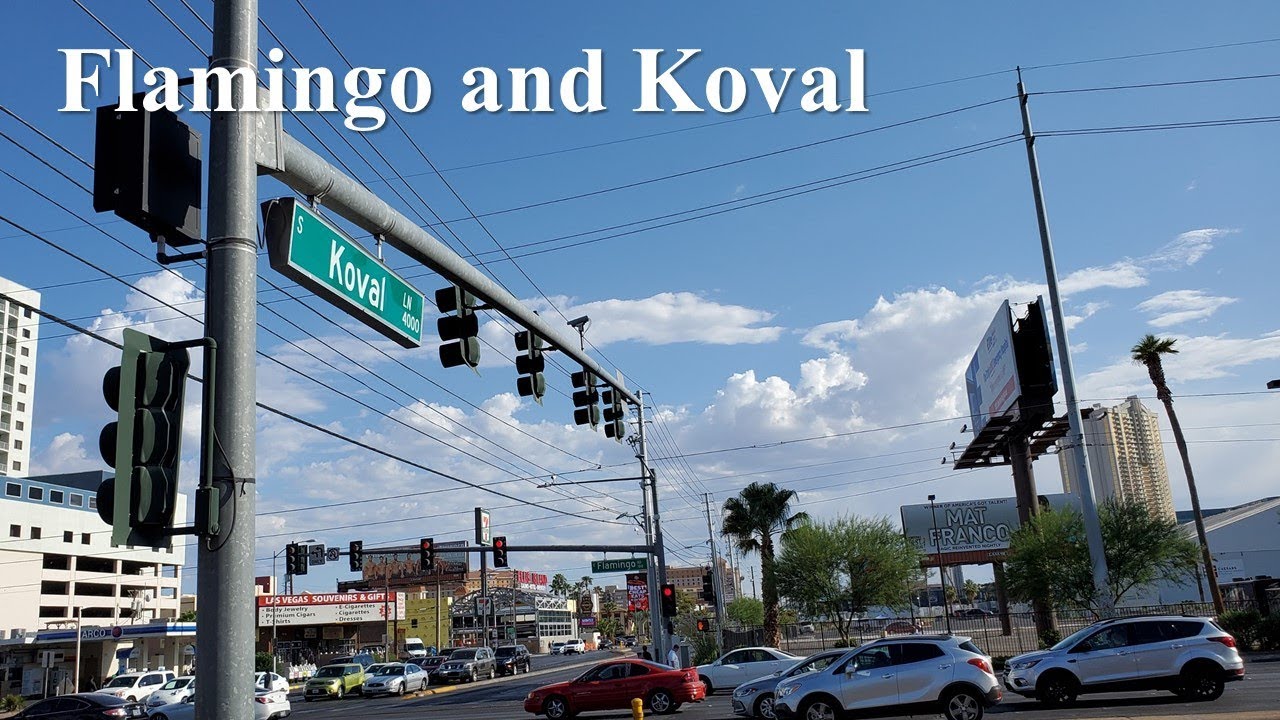This color photograph captures a bustling urban intersection in Las Vegas, Nevada, during a bright, sunny day with a few fluffy clouds scattered across the blue sky. The focal point of the image is the intersection of Flamingo Road and Coval Lane, clearly marked by the green street signs with white text. Prominently featured are the large metal utility poles with cross poles supporting multiple traffic lights. Cars approach the intersection from the right-hand side, some proceeding through on a green light while others wait at a red light in a perpendicular direction. Visible in the distance, the cross street is identified as Flamingo. The surrounding urban landscape includes a large parking garage to the left of the image, with a tall building, possibly a hotel or condominium, rising behind it. In the background, a sign for "Las Vegas Souvenirs and Gifts" can be seen, enhancing the impression of a lively, tourist-friendly area.